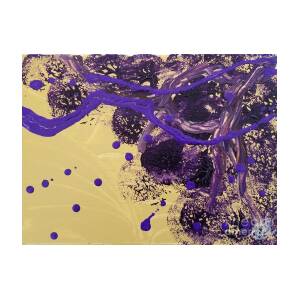The painting is a small square modern art piece dominated by chaotic and dynamic forms primarily in purple and a sand-yellow hue. The background is a matte yellow canvas, visible mostly from the bottom left to the top left, partially obscured by intricate, thick swathes and circular patterns of purple. The design features heavy, swirling purple streaks and squiggles running diagonally from the top left to the bottom right, covering much of the background along this axis. There are deep purple circular patterns dispersed throughout, with additional small purple dots and leaks spreading into the yellow areas. The upper right portion has bold purple lines with black splashes that blend with the yellow backdrop. The bottom right corner of the painting includes indecipherable white text, adding a subtle yet intriguing detail. Overall, the composition is a complex interplay of random lines, spherical shapes, and splashes, creating an abstract, modern visual experience.